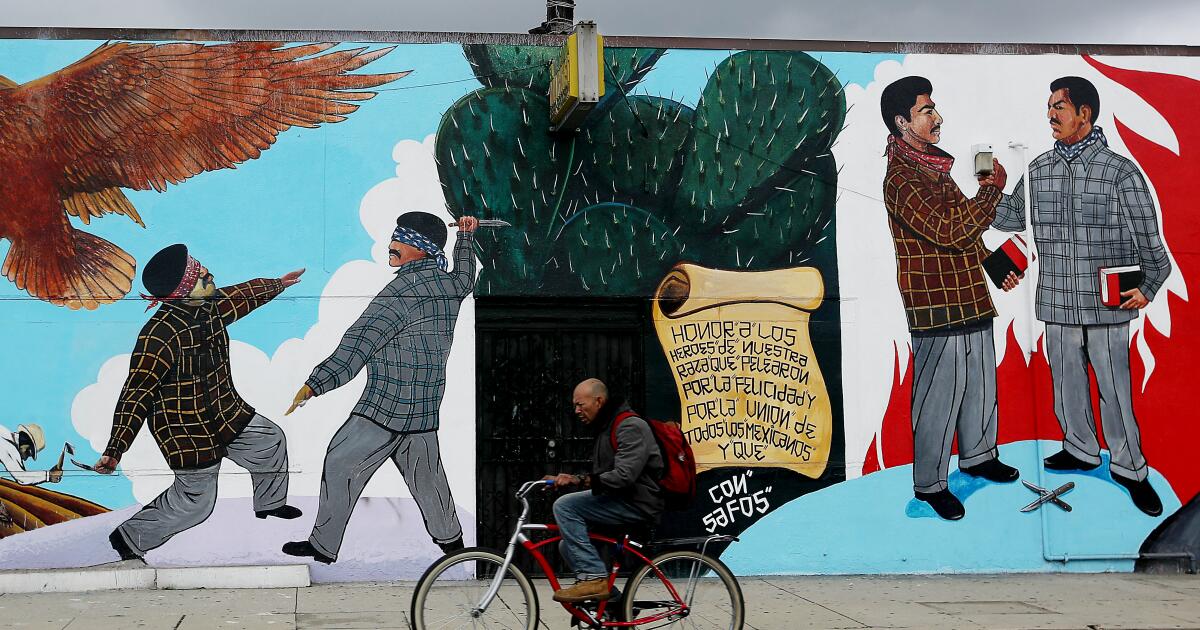The image portrays an older Black man with short gray hair riding a white and red beach cruiser bicycle down the sidewalk. He wears a gray jacket, blue jeans, tan shoes, and a red backpack. Behind him, an expansive mural stretches across a wall, displaying a vivid mix of scenes and symbols. 

The mural, towering at about 20 feet high, depicts two men on both sides; on the right, they are shaking hands, and on the left, they are fighting with knives in hand and blindfolded. The fighting duo also hold books, possibly Bibles. The background on the right is a lively red and white, while on the left, a more muted gray shade prevails. An interesting detail on the left includes an eagle’s wing in brown-orange tones. 

A second man appears on the far left, seemingly emerging from a roof with a hammer in hand. This backdrop includes elements suggesting Latino or Mexican influences, akin to the Vato LA style, with the men wearing blue or red headbands alongside plaid shirts and pants, evoking a gangbanger appearance.

Separating the two contrasting scenes of the mural is a cactus planted in the ground with thorns, portrayed in a desert motif. Below the cactus is a scroll with some writing on it, presumably in Spanish, adding an additional layer of cultural texture. The mural’s intricate detail and the man’s interaction with his surroundings create a poignant and dynamic visual narrative against the simple gray sidewalk and blue and white sky above.